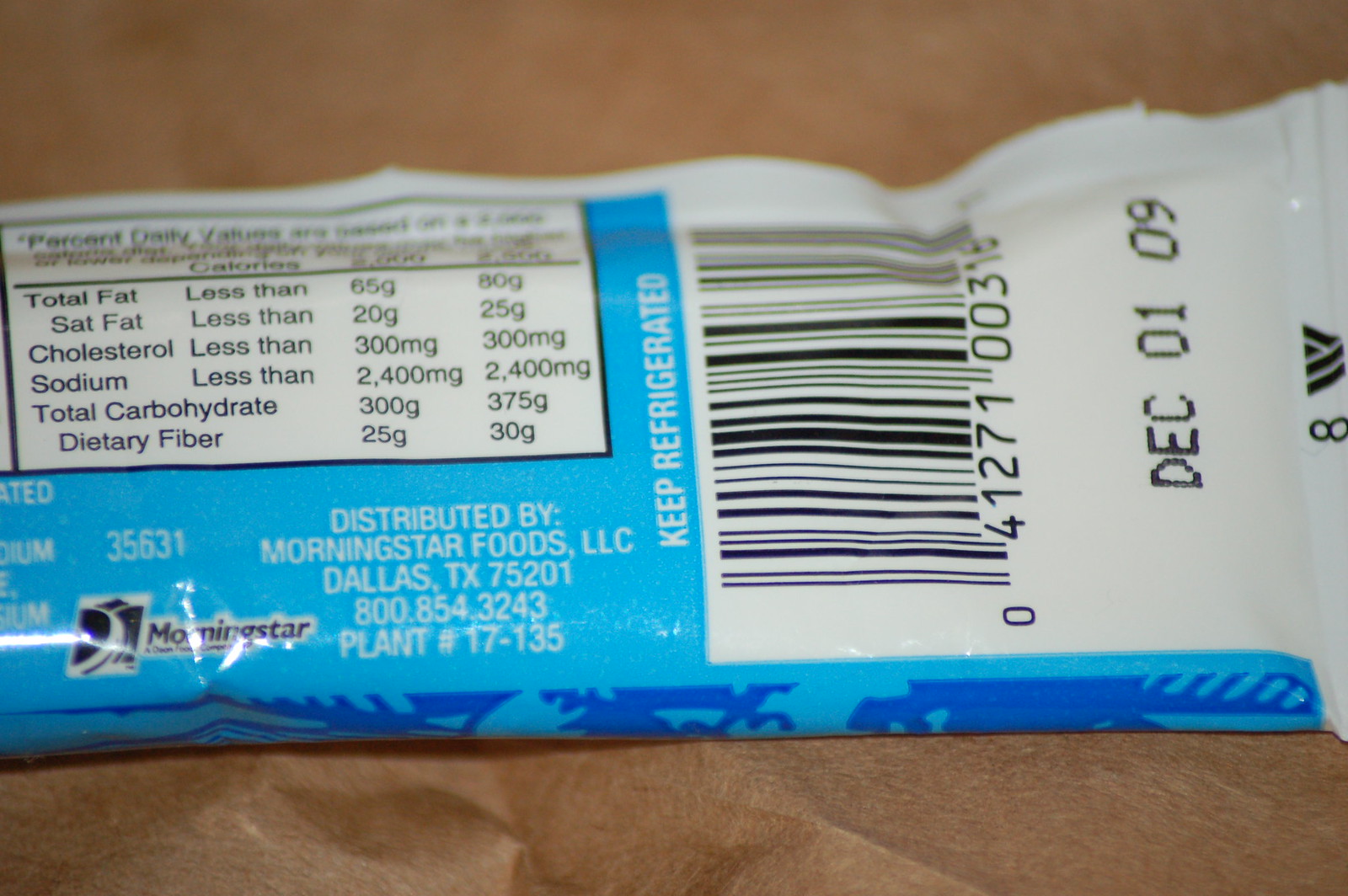The image is a color photograph taken in landscape orientation, focusing on a close-up of a food package, partially extending beyond the left edge of the frame. The packaging predominantly features light and darker shades of blue, adorned with distinct patterns. The text "distributed by Morningstar Foods, LLC, Dallas, TX 75201" is clearly printed in white on a blue background, alongside a contact number "800.854.3243". To the right, a vertically oriented barcode is visible, situated above a directive that reads "keep refrigerated." An expiry date or use-by date marked as "DEC 0109" is also noticeable near the barcode. The back of the package reveals a detailed nutrition label providing % daily values for fat (up to 65 grams), saturated fat (20 grams), cholesterol (300 milligrams), sodium (2,400 milligrams), total carbohydrates (300 grams), and dietary fiber (25 grams). Despite the detailed information, the specific identity of the food item remains undisclosed. The package appears to be set against a light brown cloth background.